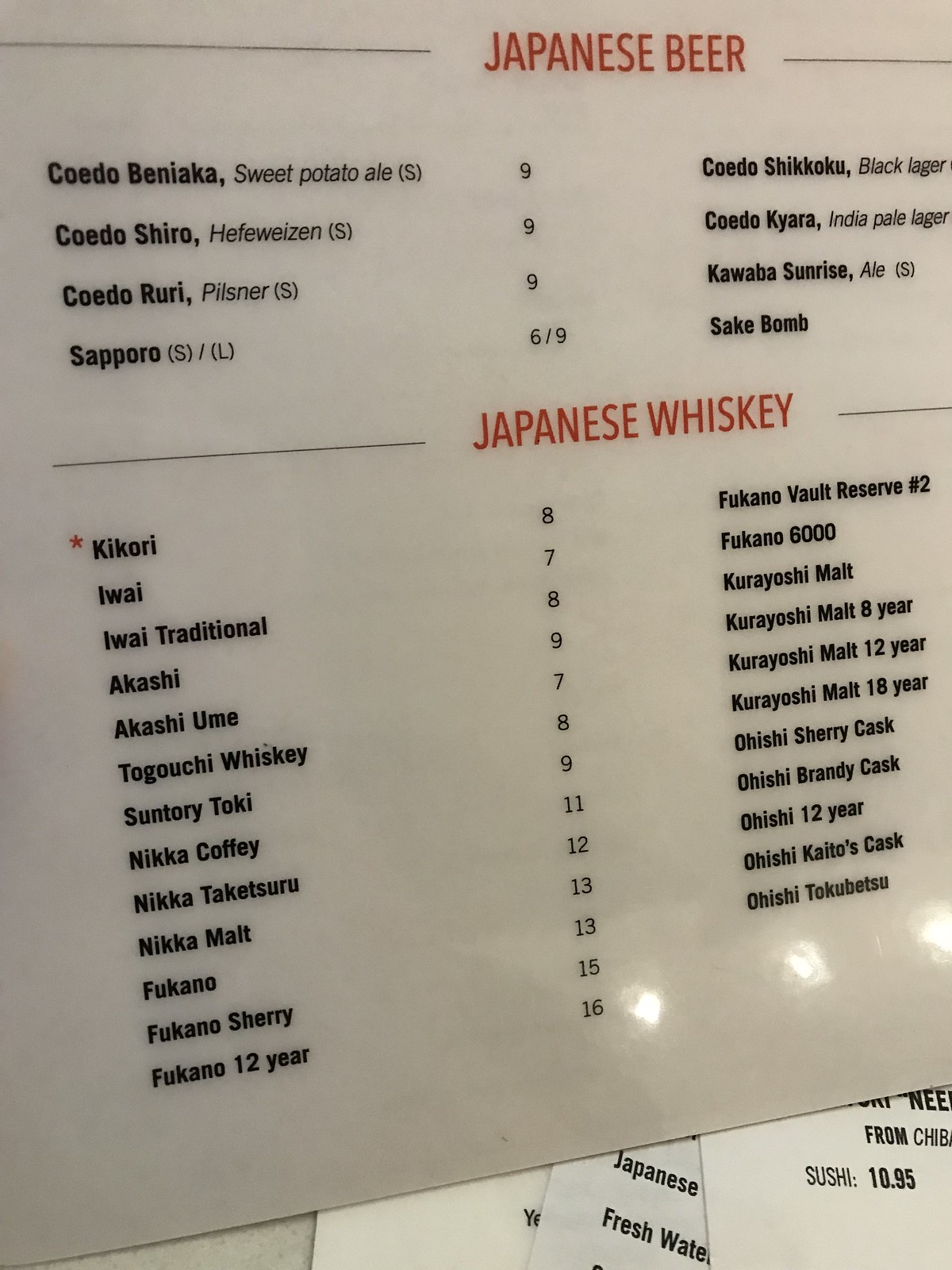The digital photograph captures a shiny, white, plastic drink menu, likely at a bar, with an organized layout and distinct red and black sections. At the top, a red line spans from the left to the center right, followed by the bold uppercase header "JAPANESE BEER" in red font. A thinner red line below this header sections off a list of various Japanese beers, written in black font. Each beer name is accompanied by its English translation and a price without a currency symbol. The beers include Sweet Potato Ale, Hefeweizen, Pilsner, Indian Pale Lager, Black Lager, and Sake Bomb.

Further down, another red line introduces the "JAPANESE WHISKEY" section in uppercase red font, separated again by a thin red line. This section lists different types of whiskey, such as Kori, Akashi, Akashi Ume, Togouchi Whiskey, Suntory Toki, Nika Coffee, and Nika Malt, each type written in black font followed by its price.

In the bottom right of the photograph, there is a background menu, much lighter in color, overlapped by the main menu. This background menu displays dark black font with partially readable items like "Japanese" and "fresh water." Additionally, a lighter printed menu lying on top features the word "sushi" and the price "10.95" in dark black print.